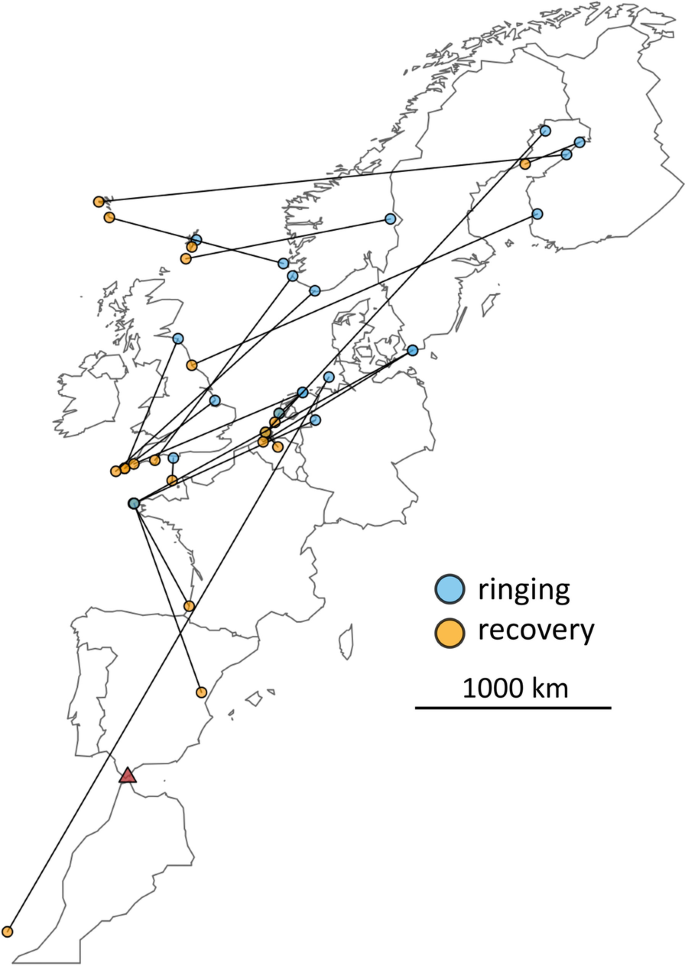The image is a detailed, simple map of several western European countries outlined in black. Each country is connected by lines leading to small, colored circles, either blue or yellow with black borders. These circles denote specific points of interest, with blue representing "ringing" and yellow representing "recovery." The lines span multiple countries, indicating connections between various locations. The bottom right corner of the map contains a comprehensive legend, explaining the meanings of the blue and yellow circles. Additionally, it includes a scale that shows a horizontal black line corresponding to 1,000 kilometers, providing a sense of distance across the mapped regions.